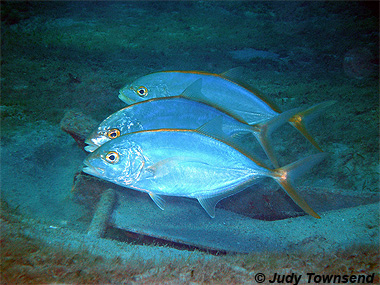This close-up underwater photograph captures three identical light to dark blue fish arranged in a perfect line, receding away from the foreground. Each fish features a distinctive golden stripe along its upper edge, extending to its bifurcated tail fin. Their eyes are yellowish with black pupils, giving them a focused appearance as they swim amidst a backdrop of greenish-blue rocks. The fish also display small orange lights on their fins, adding to their glowing blue presence.

Beneath the fish, partially obstructed by them, is a mysterious object, possibly metallic and covered in oceanic material, contributing a bluish hue. At the very bottom of the image, you can see sea foliage comprising brown and green grass or seaweed. The scene is bathed in natural underwater colors, ranging from deep blue and green to exposed gray rocks. In the bottom right corner, the photograph is marked with a copyright symbol followed by the name "Judy Townsend" in black text, confirming the creator's identity.